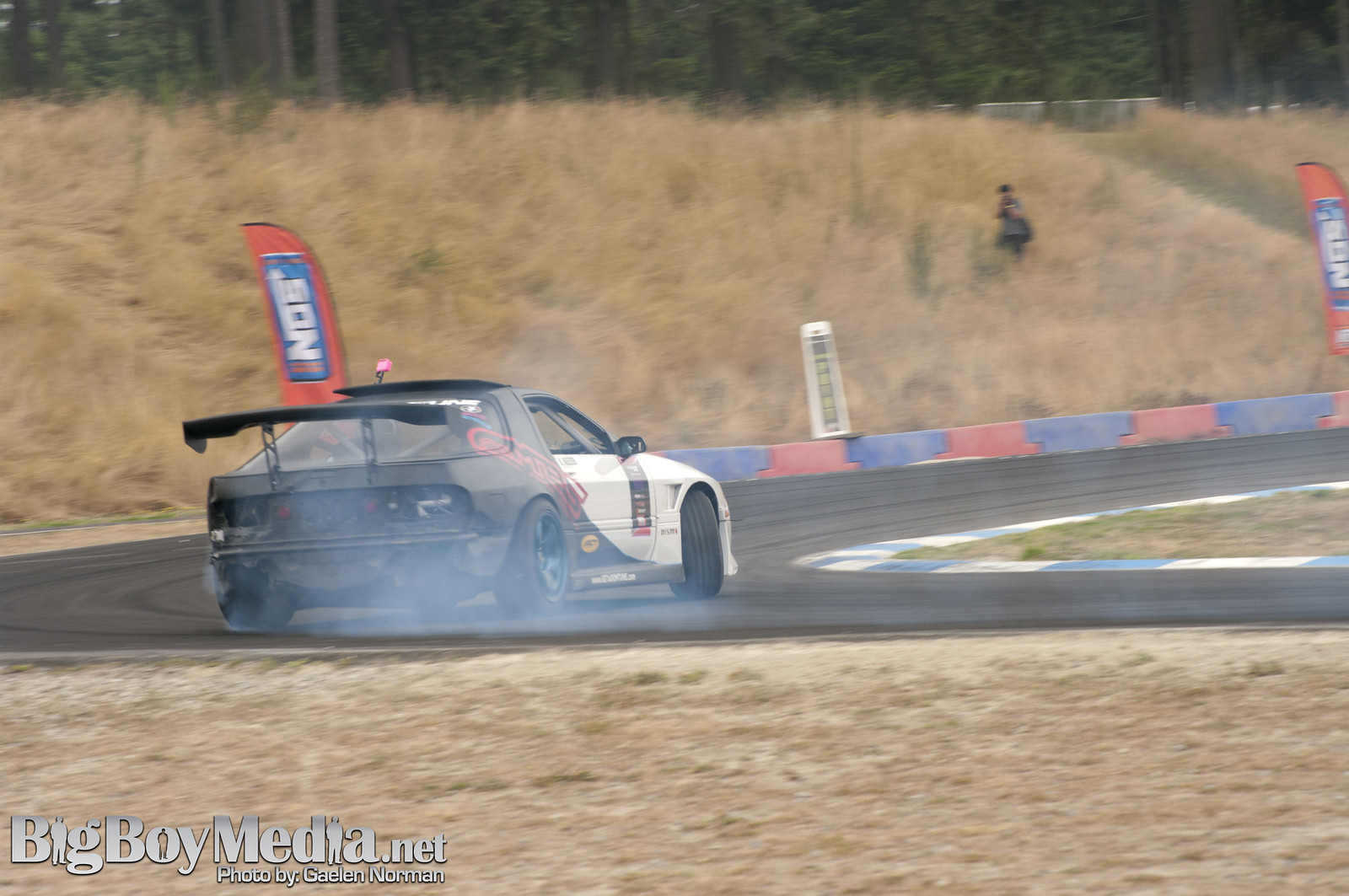This photograph captures a dynamic scene of a race car skidding around a tight curve on a rural racetrack. The racetrack is surrounded by hills covered in long, brown grass, emphasizing its rural setting. The black and white race car, adorned with a large spoiler and faint red writing visible through tire smoke, is captured in motion from a side perspective. The blacktop of the track is accentuated with a red and blue perimeter featuring sponsorship flags, notably an NOS energy drink banner. Two blurry figures stand on the distant hillside, observing the action, while another photographer is visible on the far right corner of the image. In the lower left corner, the photograph is credited to "bigboymedia.net" and attributed to Gabriel Norman in gray font.